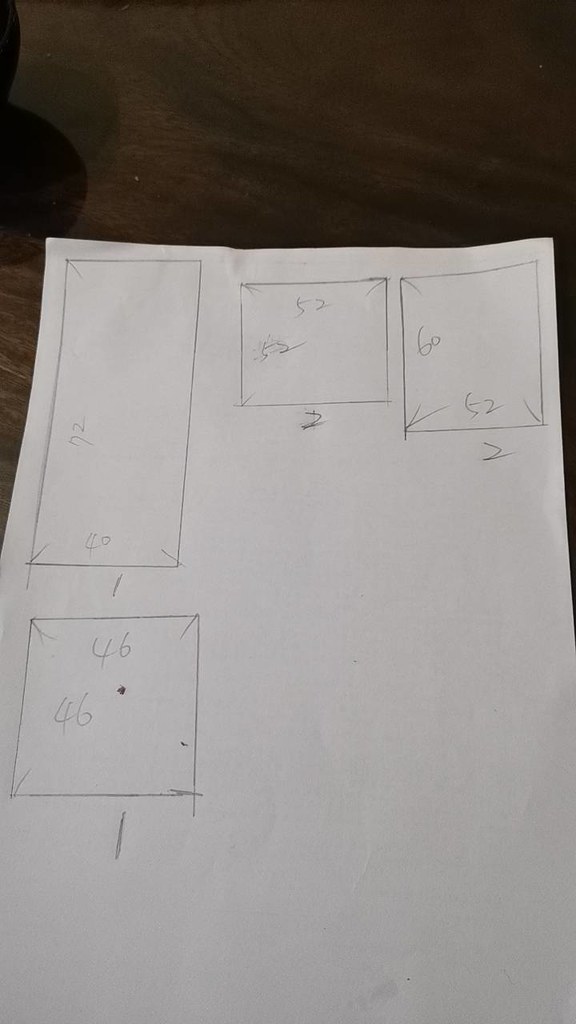The photograph showcases a piece of paper positioned on a dark wooden table, occupying about three-quarters of the image vertically. The paper features four hand-drawn geometric shapes, meticulously arranged.

- Starting at the top left and extending about halfway down the left-hand side is a long rectangle, the largest shape on the paper. It spans roughly one-eighth of the page horizontally and is annotated with dimensions "72" and "40."
- Directly beneath this rectangle is a square with labeled dimensions "46" by "46." Below this square, there is an additional line, whose purpose is unclear, potentially an error.
- In the middle of the paper's top section, there's another square marked with dimensions "52" by "52," and the number "2" positioned below it.
- On the far right side of the paper is a final square, with dimensions "60" and "52" noted alongside its sides. This shape also features the number "2" below it, similar to the middle square.

The shapes collectively form an arrangement resembling an "L" shape. The remainder of the page is blank, providing a stark contrast against the detailed annotations and shapes.